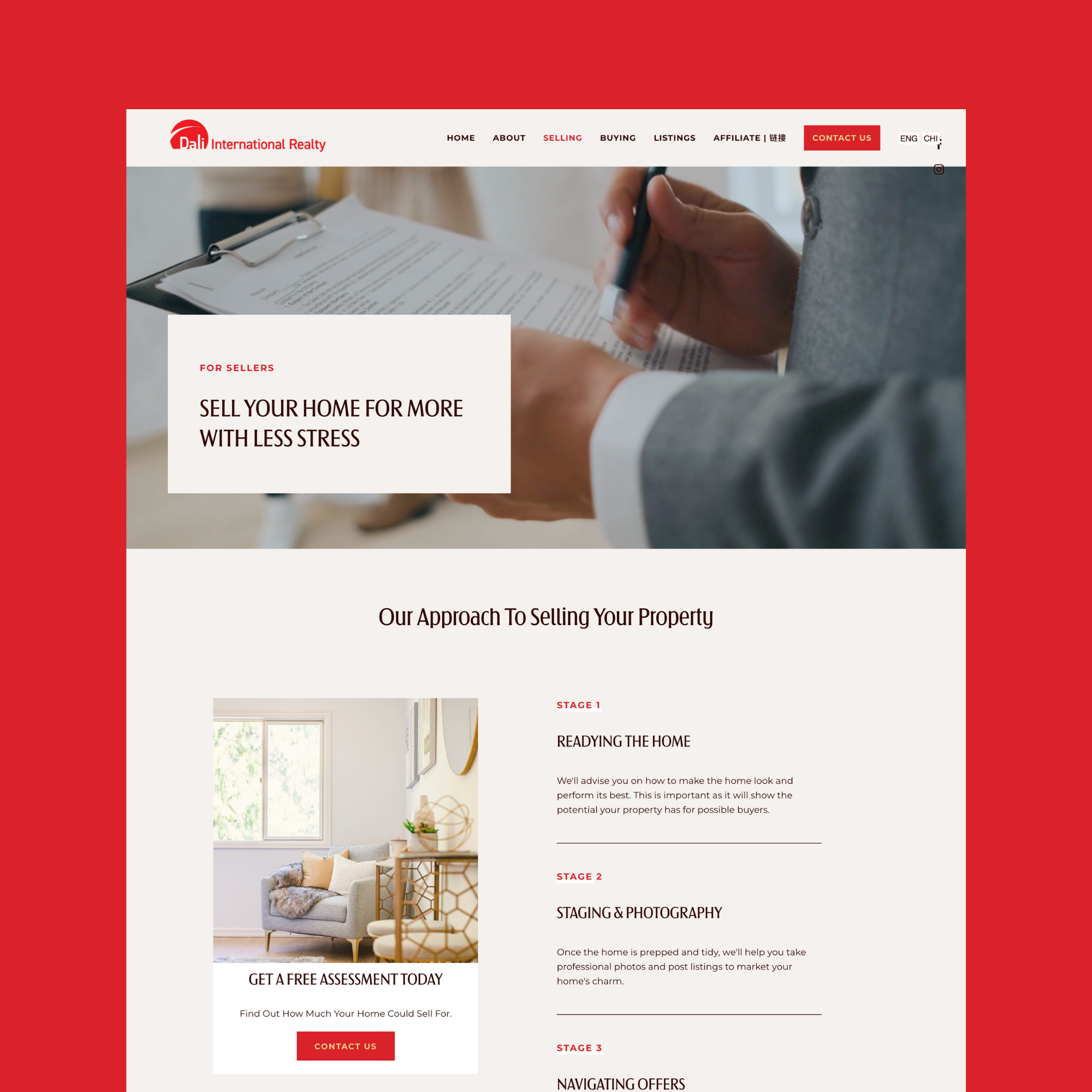On a striking red background, this image prominently features the brand "International Realty" in bold red letters, while other text is rendered in black. Key headings such as "Home," "About," "Selling," "Buying," "Listings," and "Affiliate" are clearly visible. The centerpiece of the image is a photograph of a man dressed in a suit, holding a clipboard and a pen, exuding professionalism and readiness to assist.

Adjacent to the central image, a white box outlines a streamlined approach for sellers, emphasizing how to "Sell Your Home for More with Less Stress." The steps outlined include:
- Stage One: Readying the Home.
- Stage Two: Staging and Photography.
- Stage Three: Navigating Offers.

Each stage is accompanied by detailed information, ensuring sellers understand the process.

To the left, another image presents an inviting interior of a home, with natural light streaming through an open window, symbolizing the potential and readiness for new buyers.

At the bottom of the image, a call-to-action is highlighted with a bold red rectangle that reads "Contact Us" in white, encouraging potential clients to take the next step. Additionally, the offer of a "Get a Free Assessment Today" is emphasized, providing further motivation for engagement.